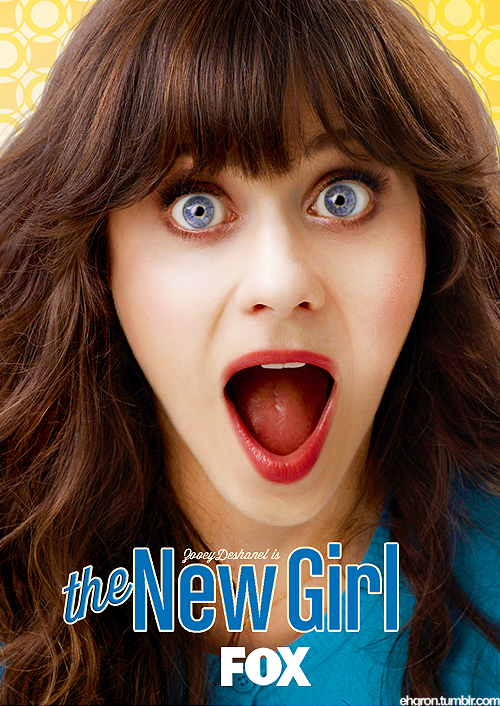The image shows a promotional poster for the show "The New Girl." The text at the bottom of the image reads "Zooey Deschanel is The New Girl," with "The New Girl" written in blue. Below this, the brand "Fox" is displayed in white in the bottom right corner, and the source website "ehgron.tumblr.com" is also visible. The poster features a young white woman with brown hair and bangs, with blue eyes wide open and a surprised expression, revealing her teeth and tongue. She is wearing lipstick and a blue dress with a button near the neck. Only her face and a portion of her shoulders are visible. The background consists of an abstract design with shades of yellow and white circular patterns.